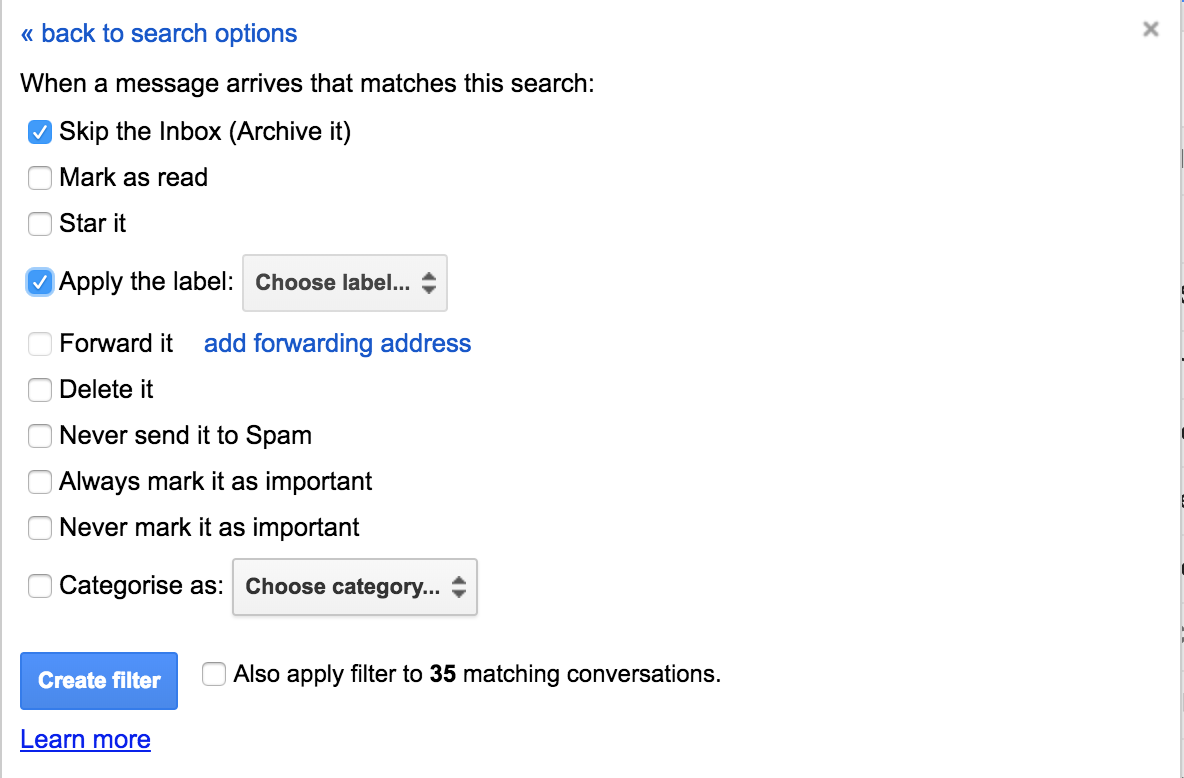The image depicts a web page with a white background. At the very top, in bright blue letters, it reads "Back to search options," accompanied by a back arrow to the left. Below, black text states, "When a message arrives that matches this search:" followed by three options: "Skip the Inbox (Archive it)," "Mark as read," and "Star it." The option "Skip the Inbox (Archive it)" is selected and highlighted in bright blue with a white checkmark inside the box.

Below these options, there is an additional setting to "Apply the label," featuring a drop-down menu inside a gray box to choose the label. Other options include "Forward it," "Delete it," "Never send it to Spam," "Always mark it as important," "Never mark it as important," and "Categorize as," with another drop-down menu for category selection. In this case, "Apply the label" is also selected and highlighted in bright blue, with a white checkmark inside.

At the bottom of these options, a bright blue button with bold white text reads "Create filter." To the right, there is a checkbox option to "Also apply filter to 35 matching conversations." Additionally, underneath that, in bright blue and underlined, it says "Learn more."